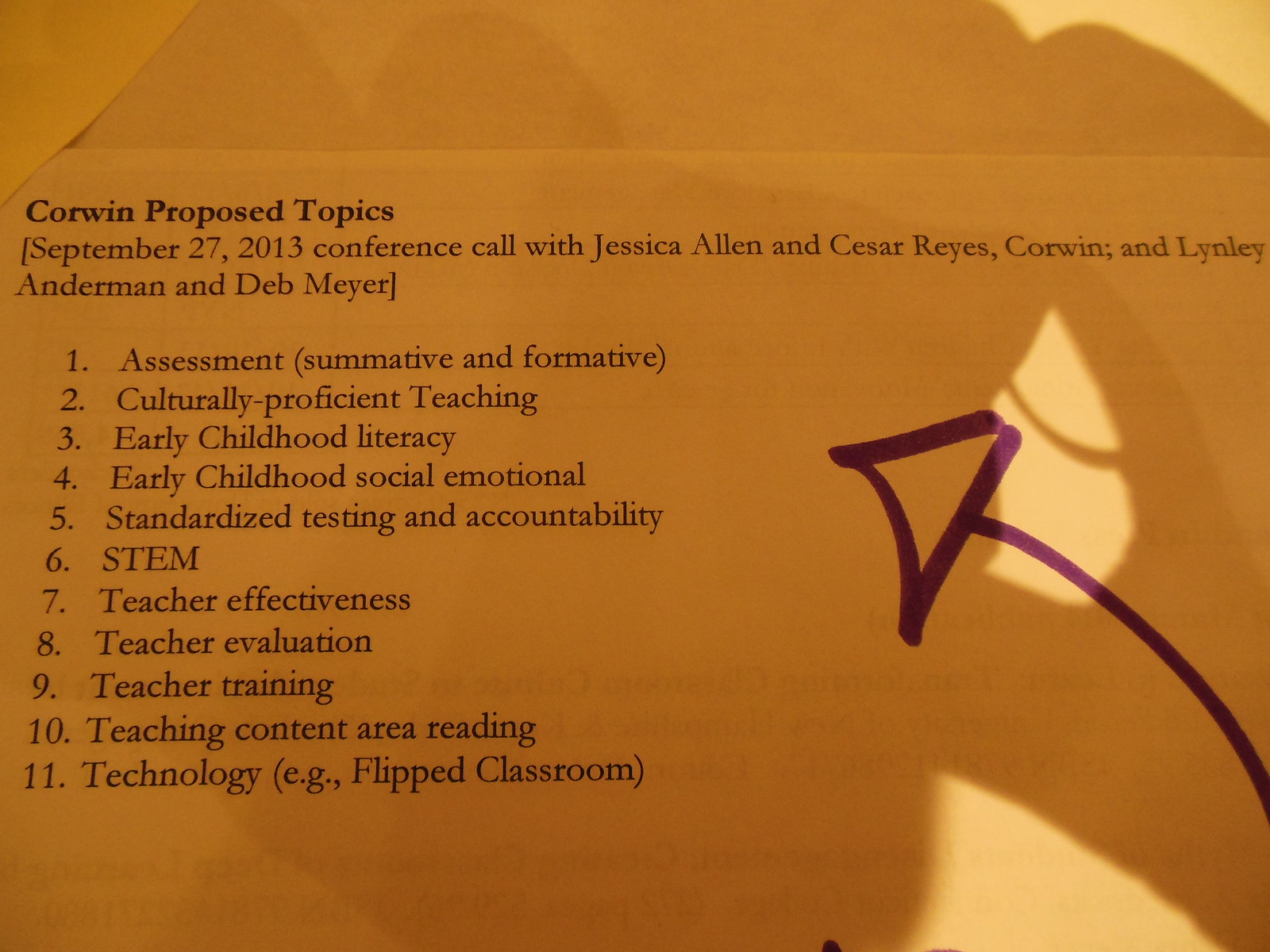The image features a detailed, landscape-oriented color photograph of a printed document on a white sheet of paper. The document is titled "Corwin Proposed Topics" and is dated September 27, 2013. It appears to be the minutes or an agenda from a conference call involving Jessica Allen, Cesar Reyes, Corwin, Lindley Anderman, and Deb Meyer. The document lists 11 discussion topics: assessment, culturally proficient teaching, early childhood literacy, early childhood social-emotional, standardized testing and accountability, STEM, teacher effectiveness, teacher evaluation, teacher training, teacher content reading, and technology, including flipped classroom models. The text is predominately black and centrally aligned on the paper, which occupies the entirety of the image. A notable feature is a hand-drawn purple arrow in the bottom right corner, pointing towards the agenda, suggesting emphasis. There is a noticeable shadow of the person taking the photograph, cast over the document, indicating the presence of strong sunlight. The photograph, rich in realism, captures both the content and context of an educational setting.